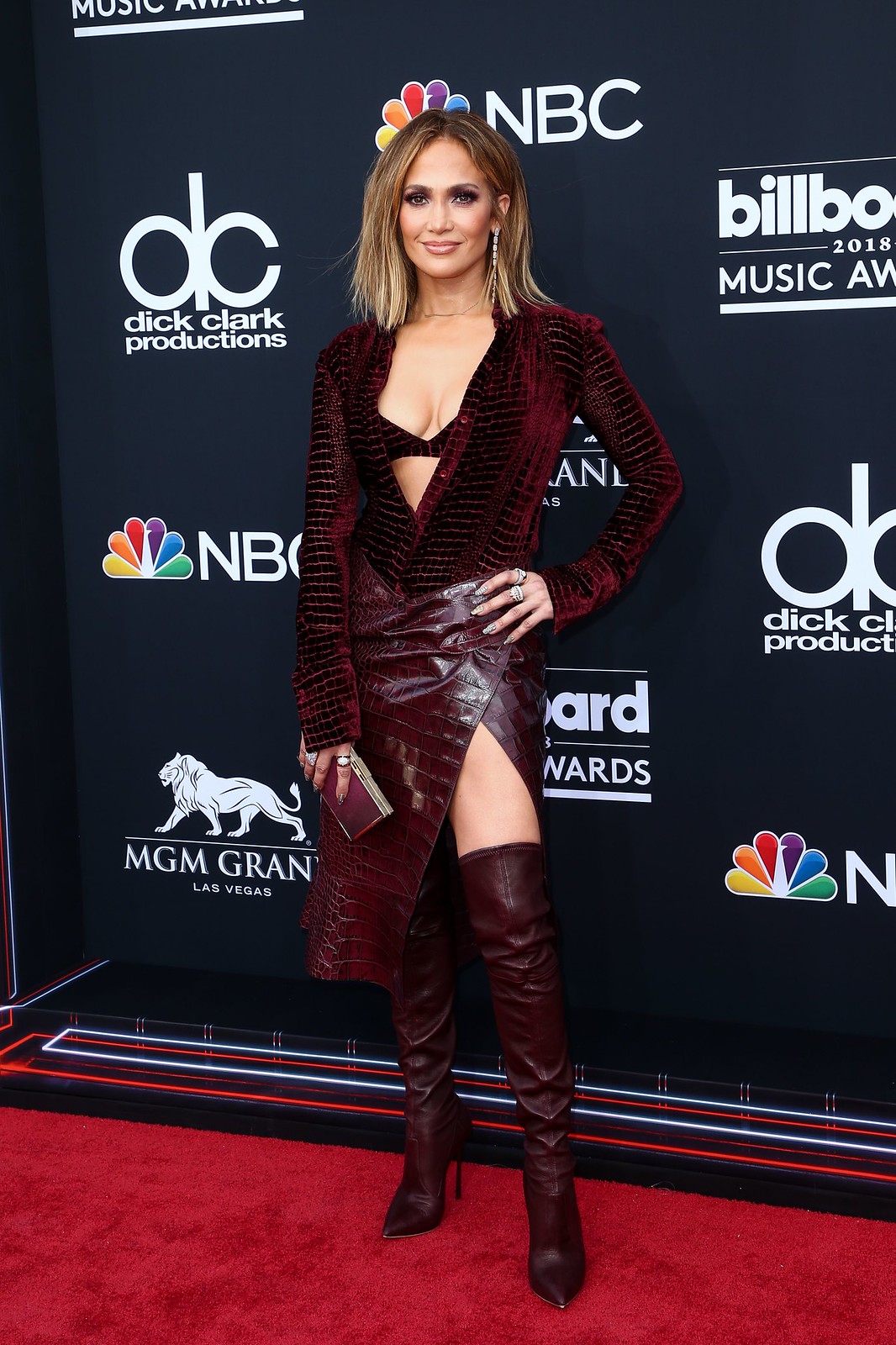Jennifer Lopez is captured posing on the red carpet at the Billboard Music Awards 2018, held at the MGM Grand in Las Vegas. She stands confidently in front of a black backdrop emblazoned with white logos of NBC, ABC, Dick Clark Productions, and other sponsors, which repeat across the wall. Jennifer's sleek shoulder-length hair features frosted blonde highlights, complementing her glamorous makeup. She dons a striking dark burgundy velvet outfit, characterized by a revealing low-cut top that exposes a matching bra, along with a side-split leather skirt. Completing her ensemble, she wears knee-high, tight, shiny burgundy boots and holds a dark red clutch in her right hand while resting her left hand on her hip.